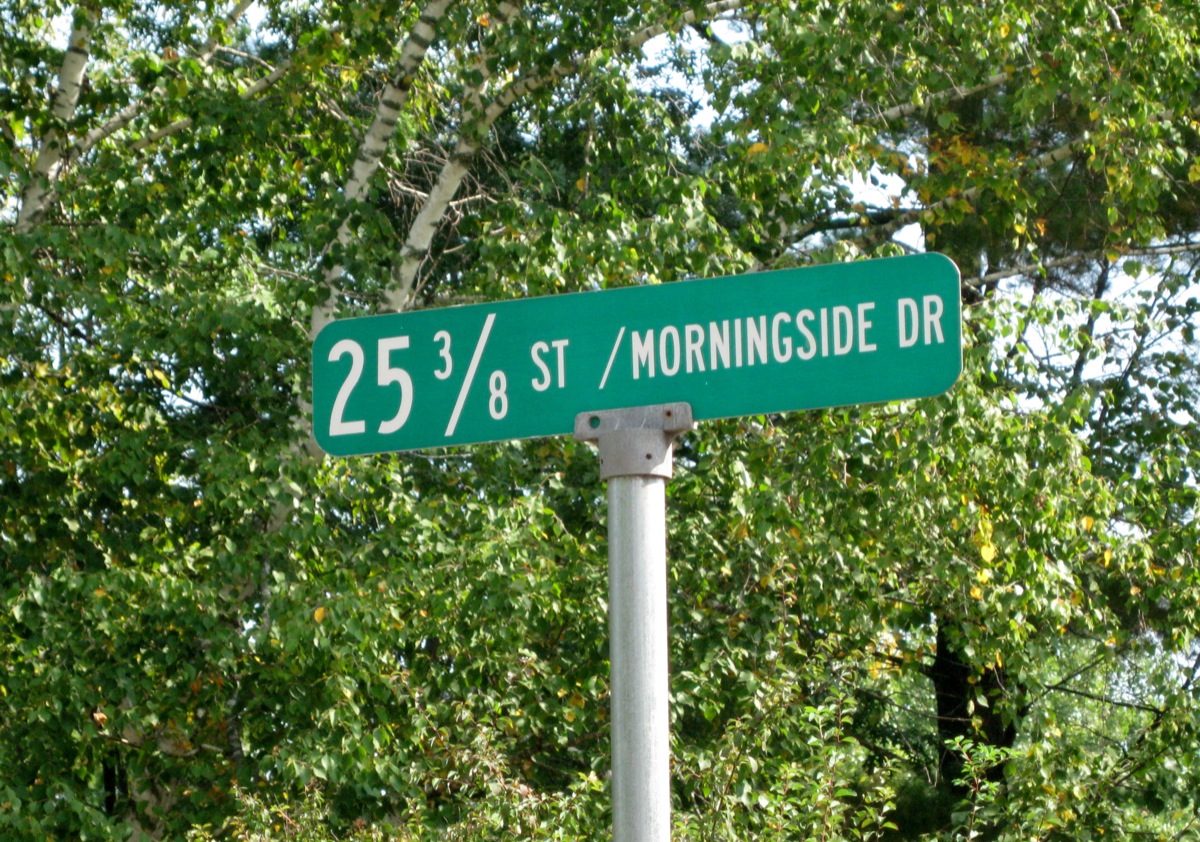The photograph depicts an outdoor scene featuring a distinct green street sign mounted on a single silver metal pole. The sign is rectangular with white lettering that reads “25-3/8 St / Morningside Drive.” The pole, positioned slightly off-center to the right at the bottom of the image, is secured to the sign by a metal clamp held in place by two bolts. The background is filled with lush greenery, showcasing healthy green leaves of various trees. Visible through the gaps in the foliage are patches of light blue sky with some clouds. The tree on the left has bark with white and darker exposed areas, while the tree on the right has darker brown or black bark. This vibrant and unusual depiction captures a surreal street name that includes a fraction, something rarely seen on typical street signs, making "25-3/8 St / Morningside Drive" notably memorable.